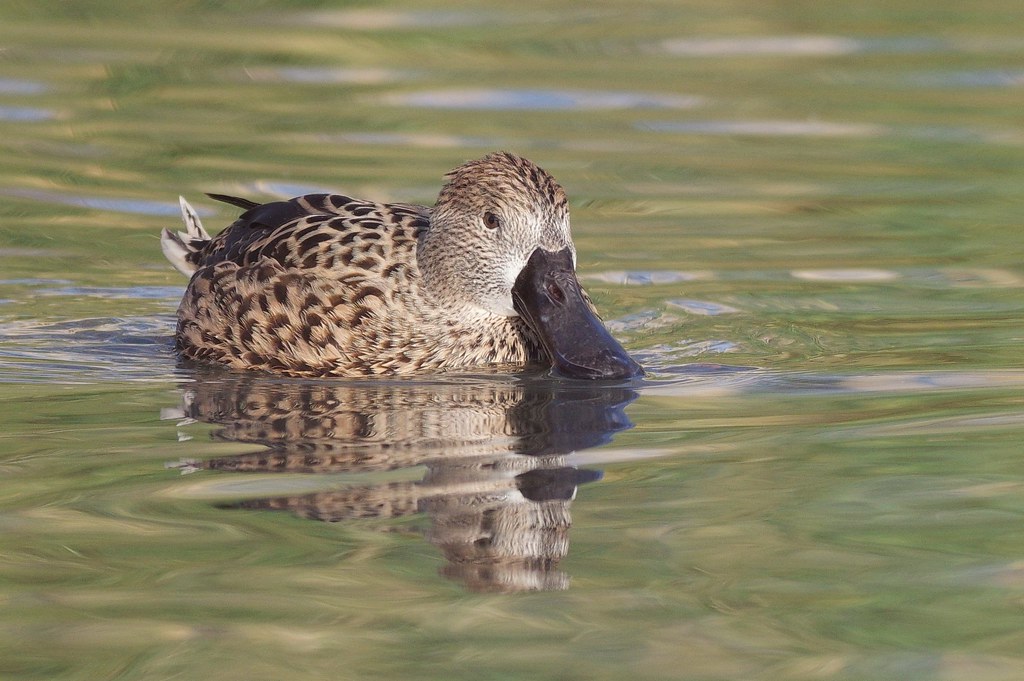This detailed outdoor photograph captures a serene lake scene dominated by a duck floating calmly in the water during daytime. The rectangular image measures approximately six inches wide by four inches high. The water, which forms the entire backdrop, is predominantly tinted green, with hints of tan and blue reflections from the sky.

Positioned towards the center left of the image, the duck is facing to the right, presenting its back end away from the viewer and its head closer. This duck has a distinctive large, flat, black bill touching the surface of the calm water. The head features cream-colored feathers with dark brown and black markings extending to the cheeks. These markings converge near its brown eye, transitioning into tan feathers with black stripes above the eye.

The duck's body showcases a complex array of colors: the back is tan with black half-circle patterns on the feathers, while the sides and neck area display a mixture of brown, light brown, white, and beige hues. The tail feathers, visible from behind, include one black feather and two cream-colored ones with dark brown interiors.

Additionally, the water reflects the duck's image, creating a mirror-like effect beneath it. The overall scene is tranquil, with slight ripples on the murky olive-green surface and occasional bluish streaks hinting at the sky above, emphasizing the peaceful and picturesque nature of the photograph.